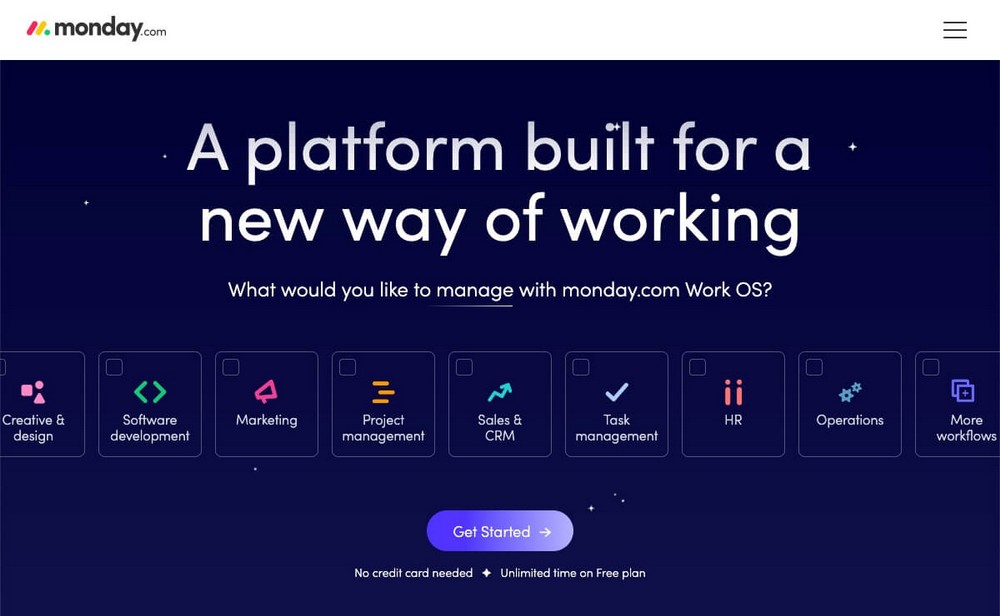This screenshot from Monday.com prominently features their distinct logo: an abstract, stylized "M" composed of a red slash, followed by a yellow slash, and concluding with a green dot. The company name, "monday.com," is displayed in lowercase letters, with ".com" aligned slightly lower. In the upper right corner of the screen, there is a hamburger menu icon.

The header section stands out with a bold purple background, overlaid with large white text flanked by small stars. The text reads: "A platform built for a new way of working. What would you like to manage with monday.com Work OS?" 

Beneath this, there are nine interactive tile boxes, each with an associated logo and title, detailing the different functionalities of the platform. The tiles include:

1. Creative and Design
2. Software Development
3. Marketing and Project Management
4. Sales and CRM
5. Task Management
6. HR
7. Operations
8. More Workflows

Each tile has a small inset square in the upper left corner, which are currently unticked.

At the bottom of this section, there is a prominent, capsule-shaped button with a gradient background that transitions from light purple to a very light shade towards the right. The button text reads: "Get Started" with a right-facing arrow. Below the button in small white text, there is a notice that reads: "No credit card needed", followed by a star, and "Unlimited time on free plan." The background is adorned with additional small stars, enhancing the visual appeal of the interface.